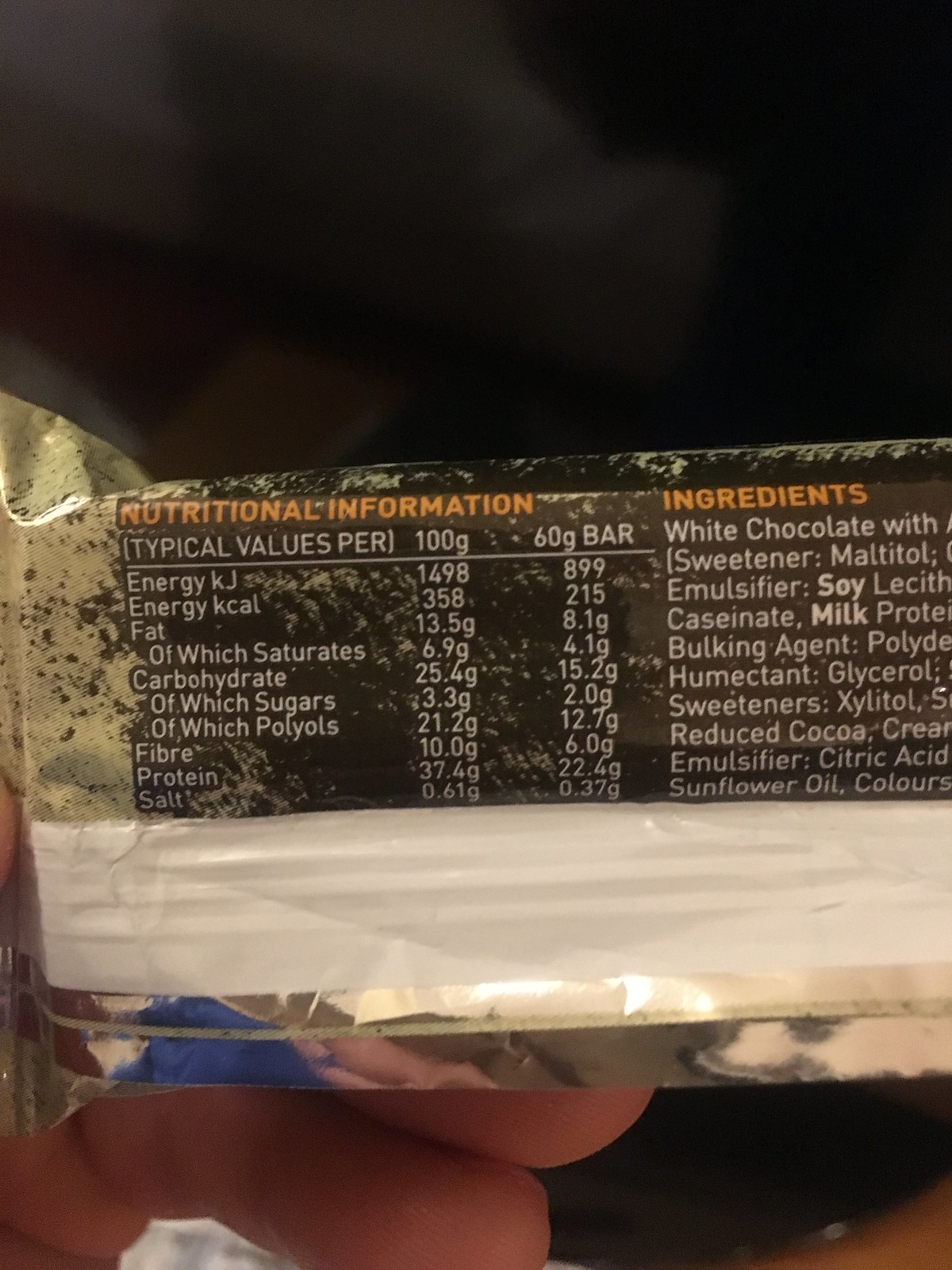The image depicts a person's hand holding a dessert item, likely a protein or energy bar, with comprehensive nutritional information and ingredients listed. The bar is brown in color, and the nutritional information is prominently displayed in orange lettering. Key nutritional values include energy measured in kilojoules and kilocalories, along with detailed information on fat, saturated fat, carbohydrates (including sugars and polyols), fiber, protein, and salt. These values are provided for both a 100-gram portion and a 60-gram bar. Ingredient details are listed to the right of the nutritional information in both orange and white letters, featuring components such as white chocolate, sweetener, emulsifier, soy lecithin, milk, bulking agent (hemikent), glycerol, xylitol, and reduced cocoa. The overall presentation suggests this is a detailed and likely non-American product, given the specific phrasing and measurement units used.